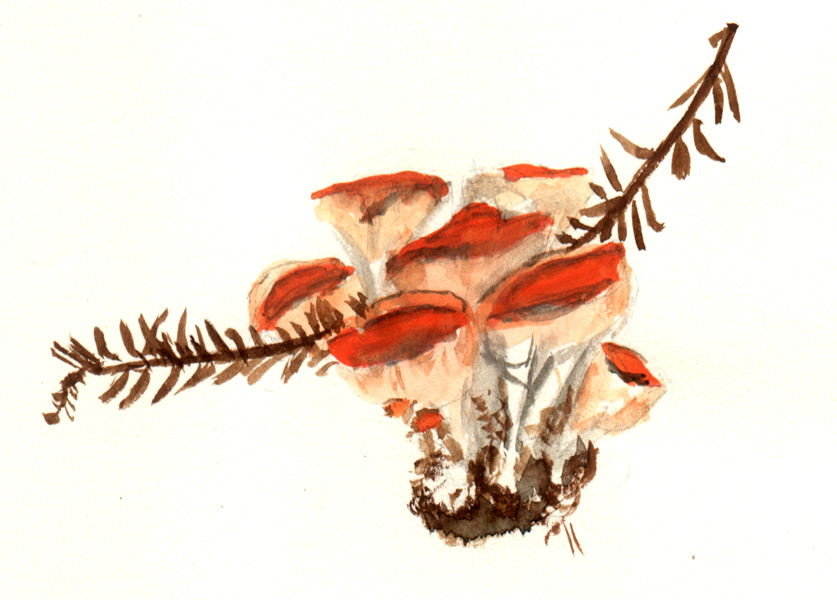This detailed watercolor painting captures a vibrant yet delicate autumnal scene featuring a cluster of mushrooms and a dormant plant. The focal point of the image is the mushrooms, which are primarily orange with some variations ranging from white to light orange. These mushrooms exhibit a diversity of shapes—some showcasing the typical mushroom cap while others are more streamlined and horizontal. They appear to either grow on or entwine with a brown branch that stretches through the composition. This branch features very small, brownish-green leaves, likely indicating a plant in late fall or early winter, evident from their lack of chlorophyll.

The painting is set on an off-white backdrop, with the bottom portion illustrating an impressionistic representation of dirt—a small, fist-sized mound of brown substance. Within this earthy base, the mushrooms rise with striking red caps, some of which flare out in a trumpet shape, adding a dash of brilliance to the natural hues. The overall scene exudes an outdoor, nature-inspired ambiance, suggesting a moment captured from a forest or woodland understory, highlighting the quiet beauty of the season's end.